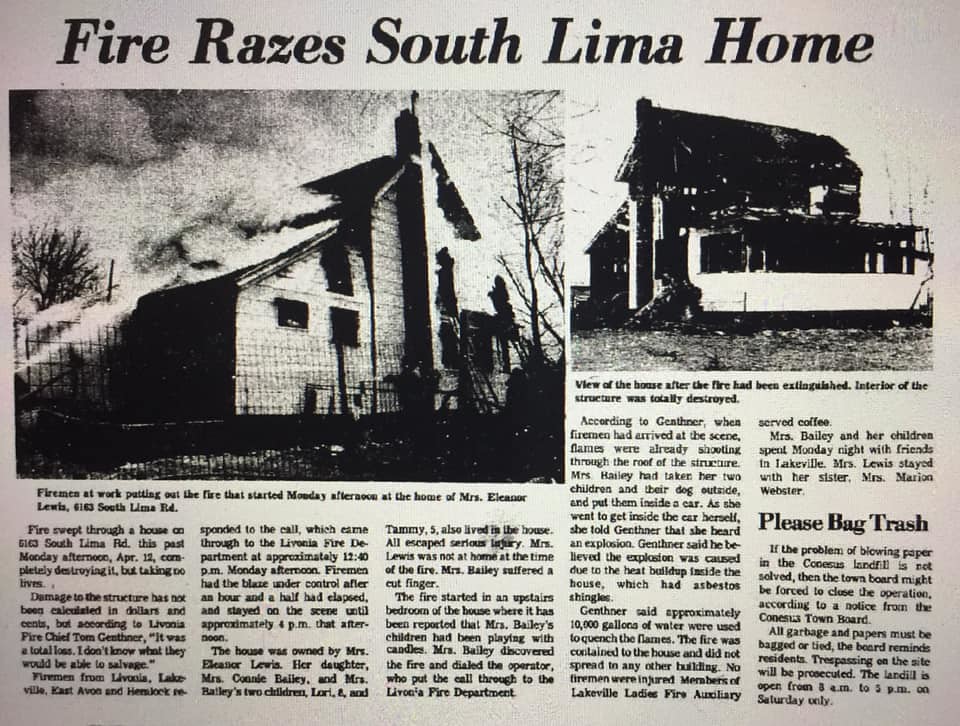The image is a scan of an older newspaper article featuring two black-and-white photos depicting the devastating effects of a fire on a house located at 5163 South Lima Road. The article, titled "Fire Razes South Lima Home," describes the event that took place on Monday afternoon, April 12th. The larger photo on the left shows the house with smoke billowing from the roof as firefighters on ladders work to extinguish the flames. The caption below this photo reads, "Firemen at work putting out the fire that started Monday." In the background, bare trees can be seen. The smaller photo on the right captures the charred remains of the house, with the caption noting, "View of the house after the fire had been extinguished; the interior of the structure was totally destroyed." According to Livonia Fire Chief Tom Centner, the house was a total loss, though fortunately, no lives were lost. Multiple fire departments including Livonia, Lakeville, Cast, Avon, and Hemlock responded to the emergency call that came through the Livonia Fire Department at approximately 12:40 PM.